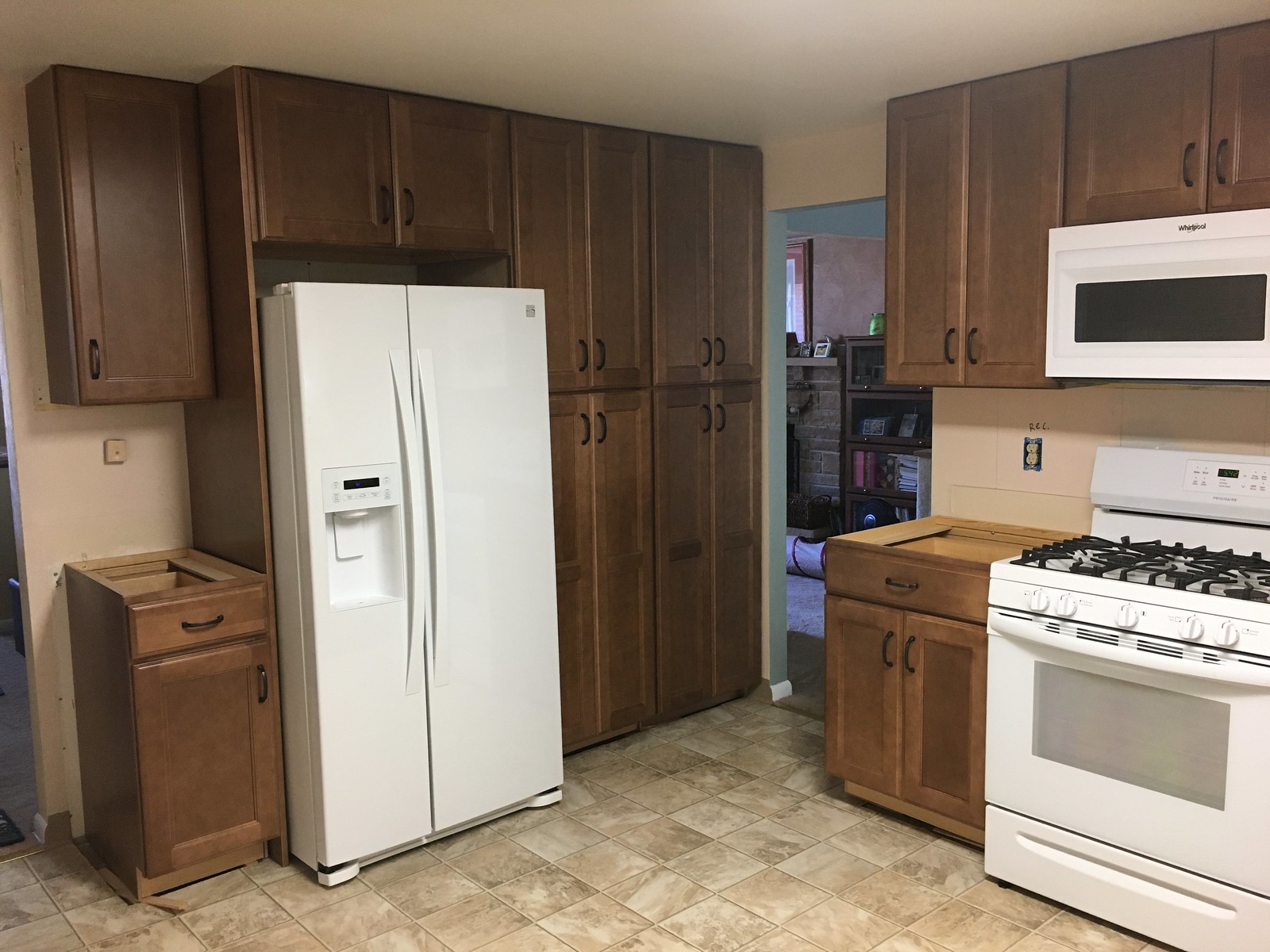This is a colour photograph of an immaculately clean, somewhat old-fashioned kitchen, with a predominantly brown and beige color palette. The kitchen features two tall, dark coffee-colored wood grain cabinets flanking a white refrigerator on the left side. Additional wood cabinets line both the left and right walls, and an electrical socket is visible above a shorter cabinet. In the lower right corner, there is a white stove with black stovetop grates, crowned by a white range hood. The floor is covered with beige, cream, and brown mottled tiles, and the walls are painted an off-white, light pink shade.

In the center of the image, a doorway leads to an adjacent room with a blue-tinged atmosphere. This room features a grey fireplace with a mirror or window above it, a bookcase, and some blue and pink objects scattered about. A rolled-up item lies on the floor, which appears to be blue. The overall scene suggests a kitchen that could be highlighted in a real estate listing due to its cleanliness and homey atmosphere.